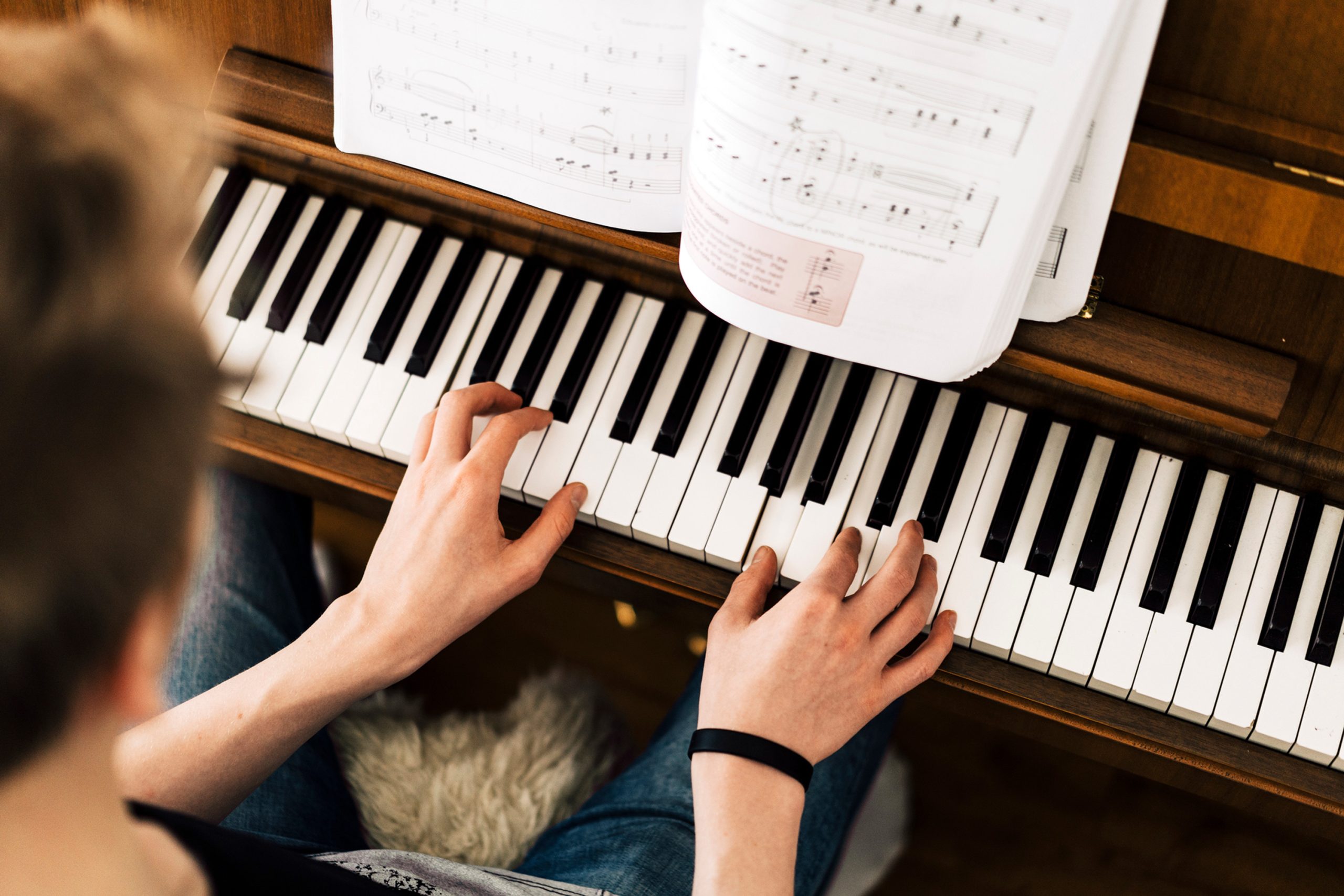This image is a photograph taken from above, capturing a young person playing a cherry wood upright piano with bright black and white keys. The individual has short brown hair and fair skin, and is wearing jeans and a black t-shirt adorned with some image, alongside a black wristband on their right wrist. Both of their hands are on the piano keys, actively pressing some of them as they play. A book of sheet music is open to the middle, propped up on the piano, showing musical notes. Notably, the right page of this book includes a pink box, indicating it may be a lesson book for practice. Between the pianist's legs, there is either a fur blanket or a dog, adding a cozy element to the scene. The person's face is out of view, focusing the attention on the act of playing and the detailed setting around them.